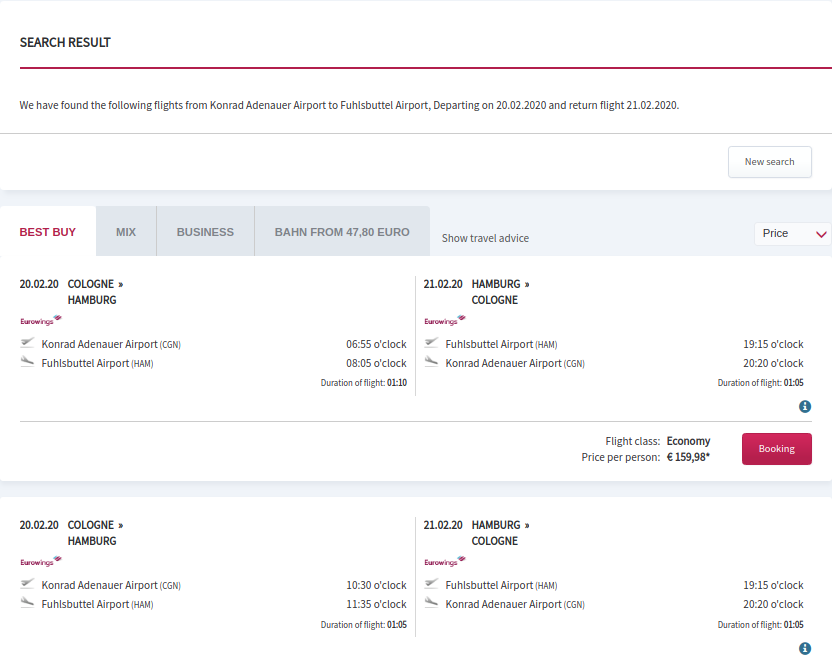On a white background, the image displays search results for flights from Conrad Adenauer Airport to FUHIS Duttel Airport, with departures on February 20, 2020, and return flights on February 21, 2020. A gray rectangle labeled "no search" is visible, indicating a lack of recent searches in that field.

Highlighted within the results is a red label "Best Buy" under the "Mixed Business" category, showing transport via a van from B-A-H-N. The cost for this transport is €47.80, with an option to "Show Travel Advice" nearby. Inside another gray rectangle, details for a flight on February 20, 2020, from Cologne to Hamburg and another for February 21, 2020, from Hamburg to Cologne are listed. Each segment contains additional unspecified information. The flight is categorized as Economy Class, with a price per person marked at €159.98.